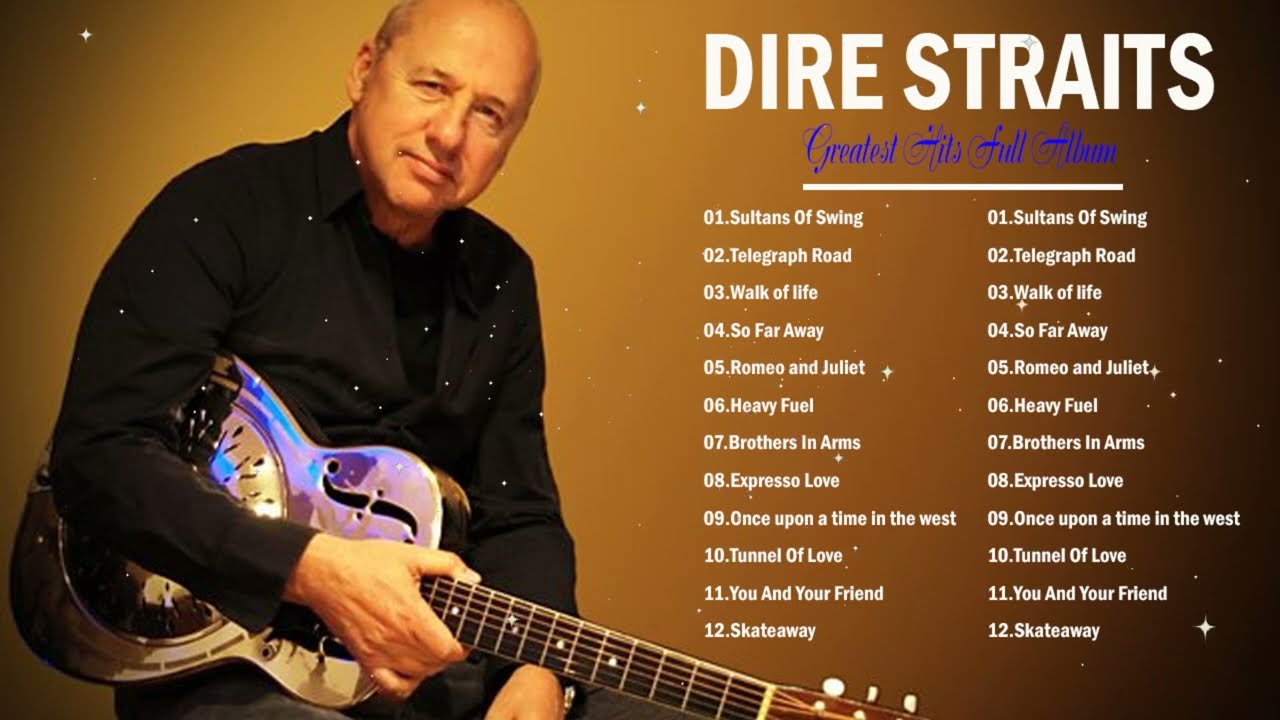The image is an advertisement for Dire Straits' "Greatest Hits Full Album." The background gradients from a golden yellow in the center to a darker, almost black vignette at the edges. On the left side of the image, a balding white man with a peaches and cream complexion is seated, wearing a black long-sleeved button-down shirt open at the collar. He holds a chrome-colored guitar with a shiny silver body and a black neck.

The text on the right-hand side features the album title "Dire Straits" in bold white capital letters, with "Greatest Hits Full Album" below it in blue cursive. Underneath are two identical vertical lists of the album's tracks in white text, including: Sultans of Swing, Telegraph Road, Walk of Life, So Far Away, Romeo and Juliet, Heavy Fuel, Brothers in Arms, Expresso Love, Once Upon a Time in the West, Tunnel of Love, You and Your Friend, and Skateaway. The lists are inexplicably repeated side by side, each numbered from 1 to 12.